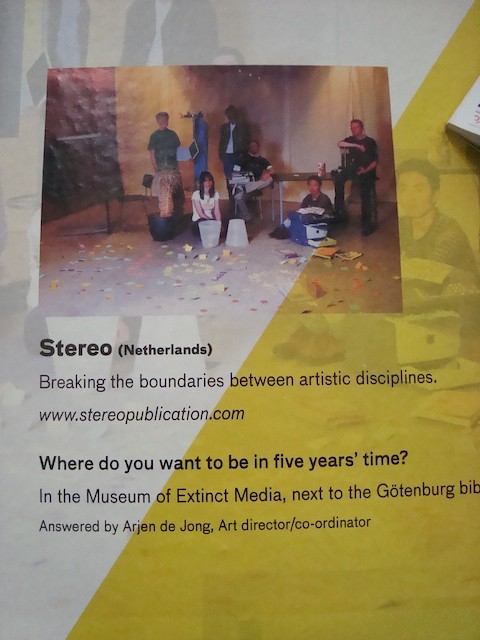The vertically aligned rectangular image is a poster featuring a central photograph of six people engaging in an activity on the ground. In the foreground of this photograph, a woman is seated on the left next to an upright bucket, with an upside-down bucket nearby, while a man sits on the right. In the background, there are two people seated at a table – one on the upper right and another on the left side of the table – along with two men standing. The ground is scattered with colorful items resembling confetti or post-it notes. 

Beneath this image, bold black text states, "Stereo (Netherlands): Breaking the boundaries between artistic disciplines," followed by the website, www.stereopublication.com. The poster includes a question, "Where do you want to be in five years’ time?" with an answer, "In the Museum of Extinct Media, next to Gothenburg," which is attributed to Arjun Dejong, art director/coordinator. The colors visible in the poster are yellow, white, black, brown, light brown, light blue, and dark blue, suggesting a dynamic and multifaceted composition suitable for a classroom display.